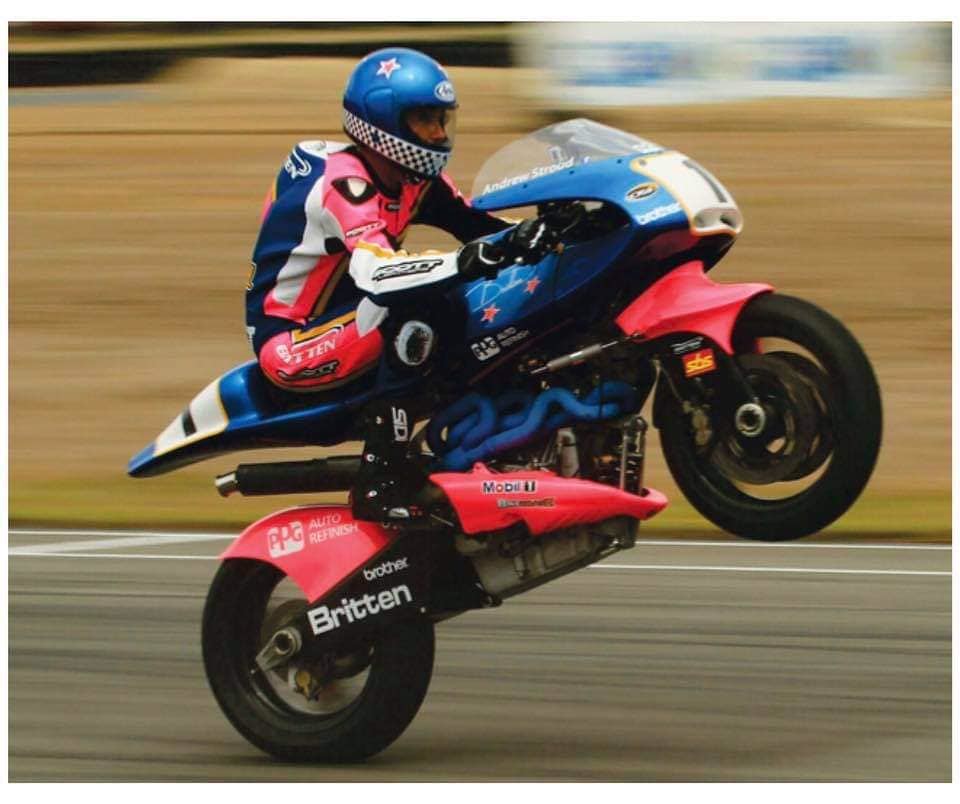This image captures the dynamic side profile of a man mid-wheelie on a decorated motorcycle during a race, evidenced by his race helmet and the bike's adorned graphics. The motorcycle itself, sporting red, white, and blue colors, prominently features advertisements including "Mobile Gasoline," "Brother Britain," and "PPG Auto Refinish." The windscreen reads "Andrew Stroud" in white lettering. The rider, matching his bike's colors, wears a blue helmet with a striking red star and black and white trim. The image is taken while in motion, giving it a blurred background that accentuates the action.